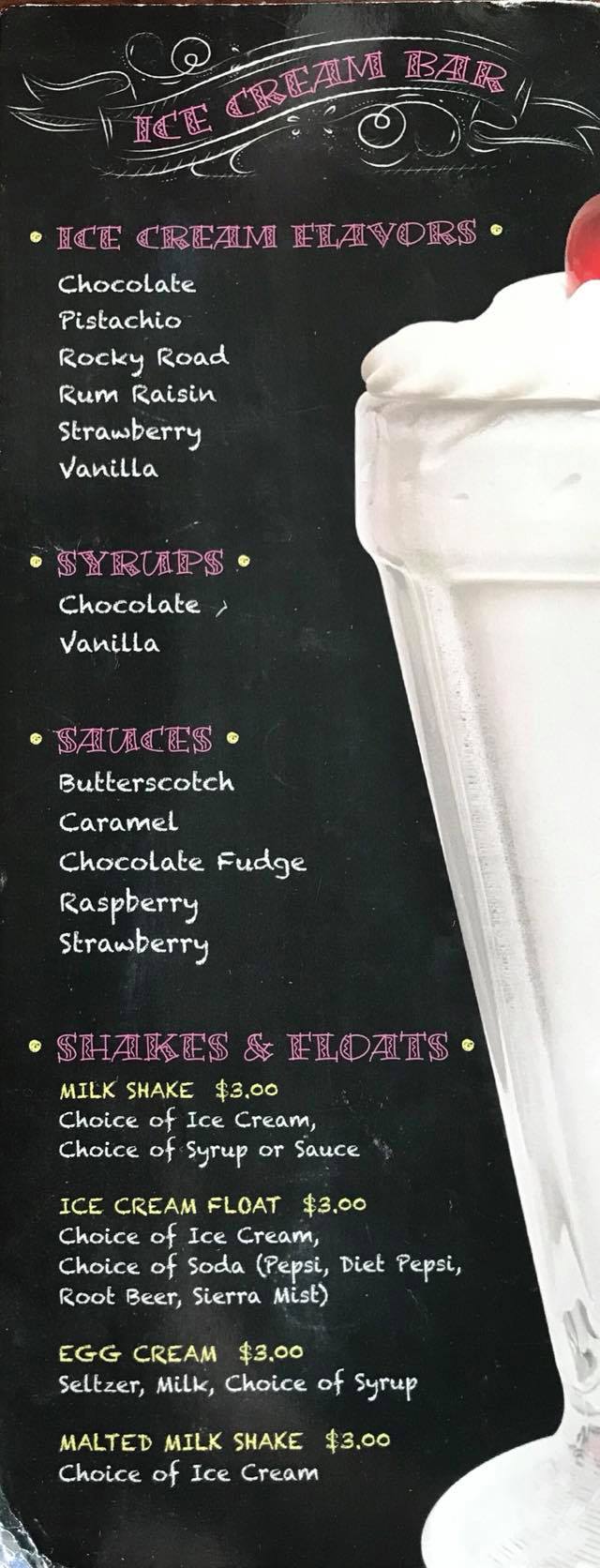**Captivating Advertisement for an Ice Cream Shop**

Against a sleek black background, this eye-catching advertisement for an ice cream shop is splashed with vibrant pink, purple, yellow, and white text. At the top, *"Ice Cream Bar"* is prominently displayed in a captivating purple-pink hue, framed by a delicate white ribbon graphic. Below, in pink-purple text, the offerings begin with *"Ice Cream Flavors,"* followed by a list of tempting choices in white: Chocolate, Pistachio, Rocky Road, Rum Raisin, Strawberry, and Vanilla.

Further down, the ad features *"Syrups"* in purple, with options listed in white: Chocolate and Vanilla. Continuing, *"Sauces"* in purple introduces a mouth-watering selection in white: Butterscotch, Caramel, Chocolate Fudge, Raspberry, and Strawberry.

The next section, labeled *"Shakes & Floats"* in purple, includes enticing menu items in yellow. *"Milkshake – $3"* allows for a choice of ice cream and syrup or sauce. The *"Ice Cream Float – $3"* offers a delicious combination of ice cream and soda, with options like Pepsi, Diet Pepsi, Root Beer, and Sierra Mist. Additionally, *"Ice Cream Soda – $3"* highlights a mix of ice cream, milk, and syrup.

The final treat featured is the *"Malted Milkshake – $3,"* providing a nostalgic option with a choice of ice cream. To the right of the text, a side profile of a tall, elegant glass showcases creamy, white ice cream crowned with a slightly obscured red cherry, adding a touch of classic dessert charm to the advertisement. 

This visually appealing poster effectively communicates a variety of delectable treats, enticing customers with its detailed and colorful layout.